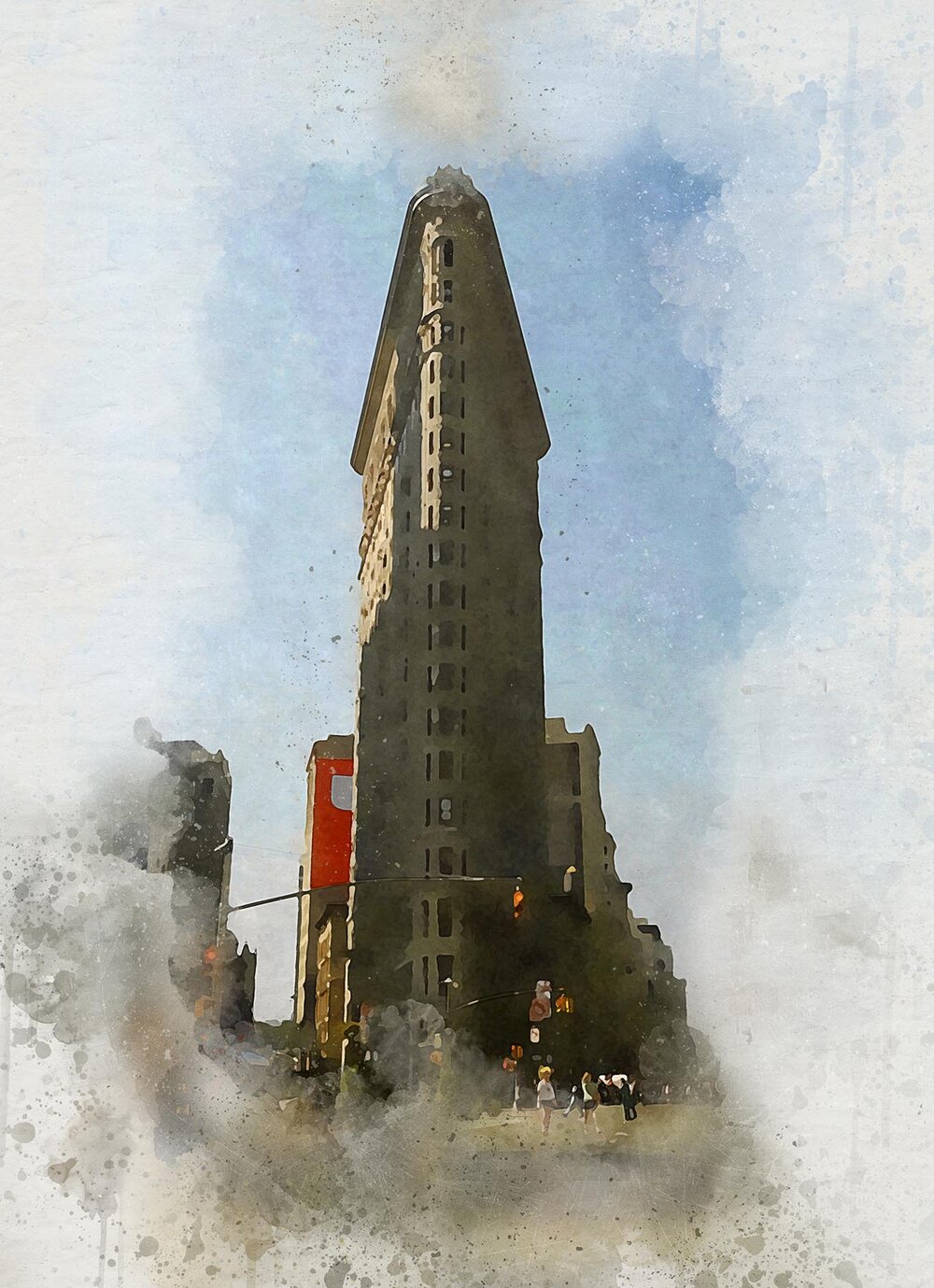The image is a detailed painting, likely a watercolor or mixed medium, of the iconic Flatiron Building in New York City. The building is a very tall, narrow, and triangular-shaped skyscraper, prominent in the center of the artwork. It has a dark gray or clay-like color with multiple windows. The painting features a blue sky with white clouds, and the edges of the painting fade into cloud-like dust, creating a vignetted effect. Below the building, there are people walking along the street, and a prominent traffic light in front of the building displays a red light. Further back, there are additional buildings that are significantly shorter than the Flatiron, one of which has a large red and white billboard. The overall composition emphasizes the towering presence of the Flatiron Building while incorporating atmospheric elements that blend into abstract brushstrokes and speckles, creating a seamless transition from the detailed center to the faded edges.